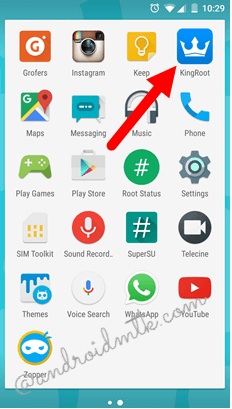The screenshot depicts a cell phone home screen featuring a neatly organized grid of apps set against a teal blue border. At the top of the screen, various status icons are displayed: an alarm clock, a Wi-Fi signal, a speaker volume icon, and a nearly depleted battery indicator, with the time reading 10:29. A watermark at the bottom of the image reads "androidmtk.com."

The home screen layout consists of four columns of apps spanning five full rows and an additional row containing a single app. A prominent red arrow at the center of the image points upward to the "King Root" app, which is marked by a blue and white crown logo. 

Here is the complete list of apps as they appear from top to bottom and left to right:
- Groofers
- Instagram
- Keep
- King Root
- Maps
- Messaging
- Music
- Phone
- Play Games
- Play Store
- Root Status
- Settings
- Sim Toolkit
- Sound Record
- SuperSU
- Telcline
- Themes
- Voice Search
- WhatsApp
- YouTube
- Zooper

Below the grid structure, there are two white indicator dots, likely representing additional home screens.